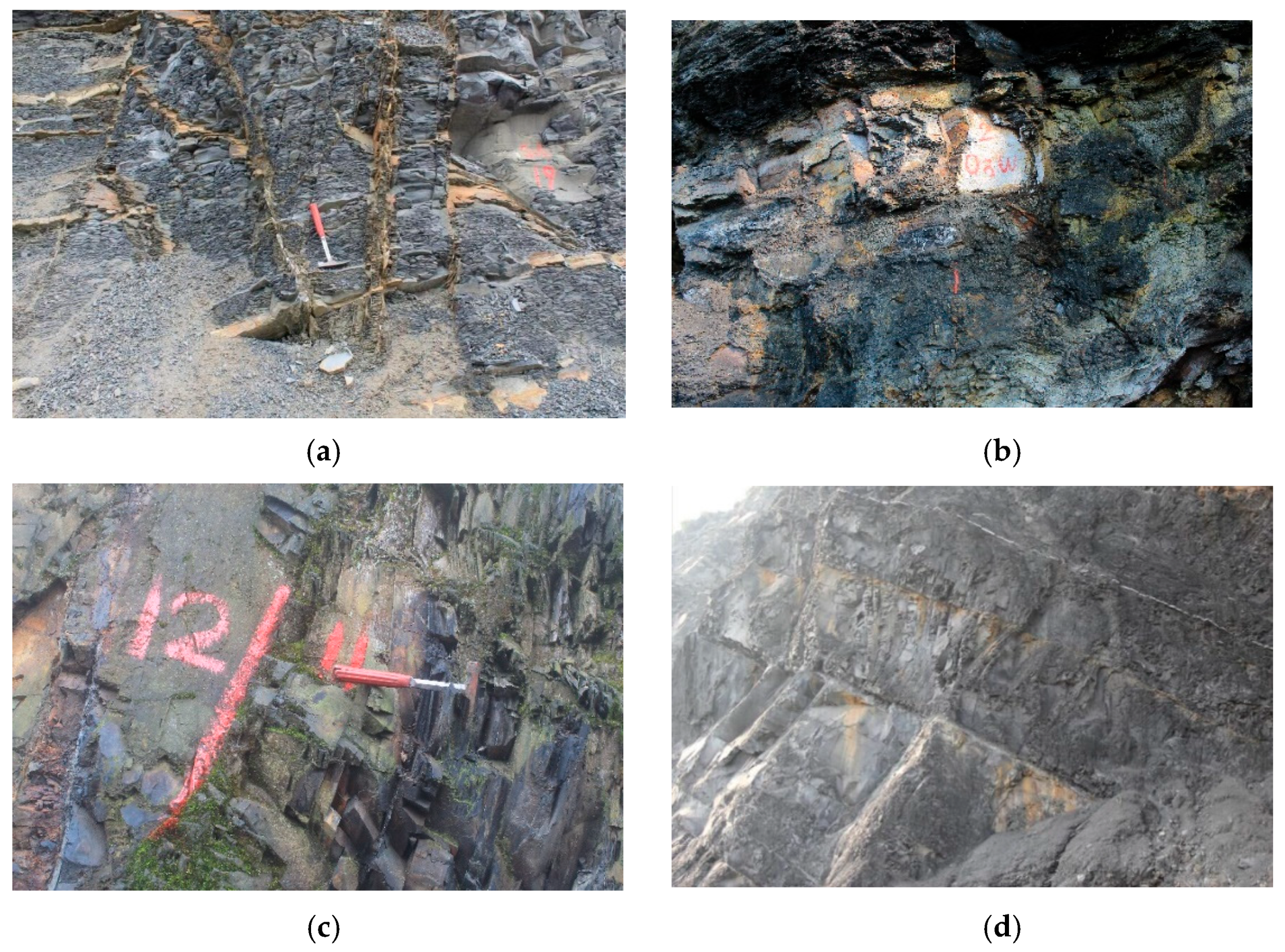The block of four images, labeled A, B, C, and D, likely found in an educational or archaeological context, display a series of rock or mountain surfaces with varying details. Image A features a rocky ground with gray and brown tones, and prominently shows a small pickaxe with a red handle and silver head placed against the rock surface. Image B provides an up-close view of a darker rock wall marked with what appears to be white chalk or spray paint indicating "202W." This rocky surface is heterogeneous with shades of brown, black, green, and gray. Image C showcases a jagged rock wall with hues of black, green, and gray, and is marked with red paint displaying "12/" followed by numbers that are partially obscured. Another red-handled tool is visible here. Finally, image D presents a rugged, steep rock face composed of black, brown, and gray rocks, but with no visible markings. Each image offers a detailed look into the textures and markings relevant to what might be an archaeological dig or geological survey.